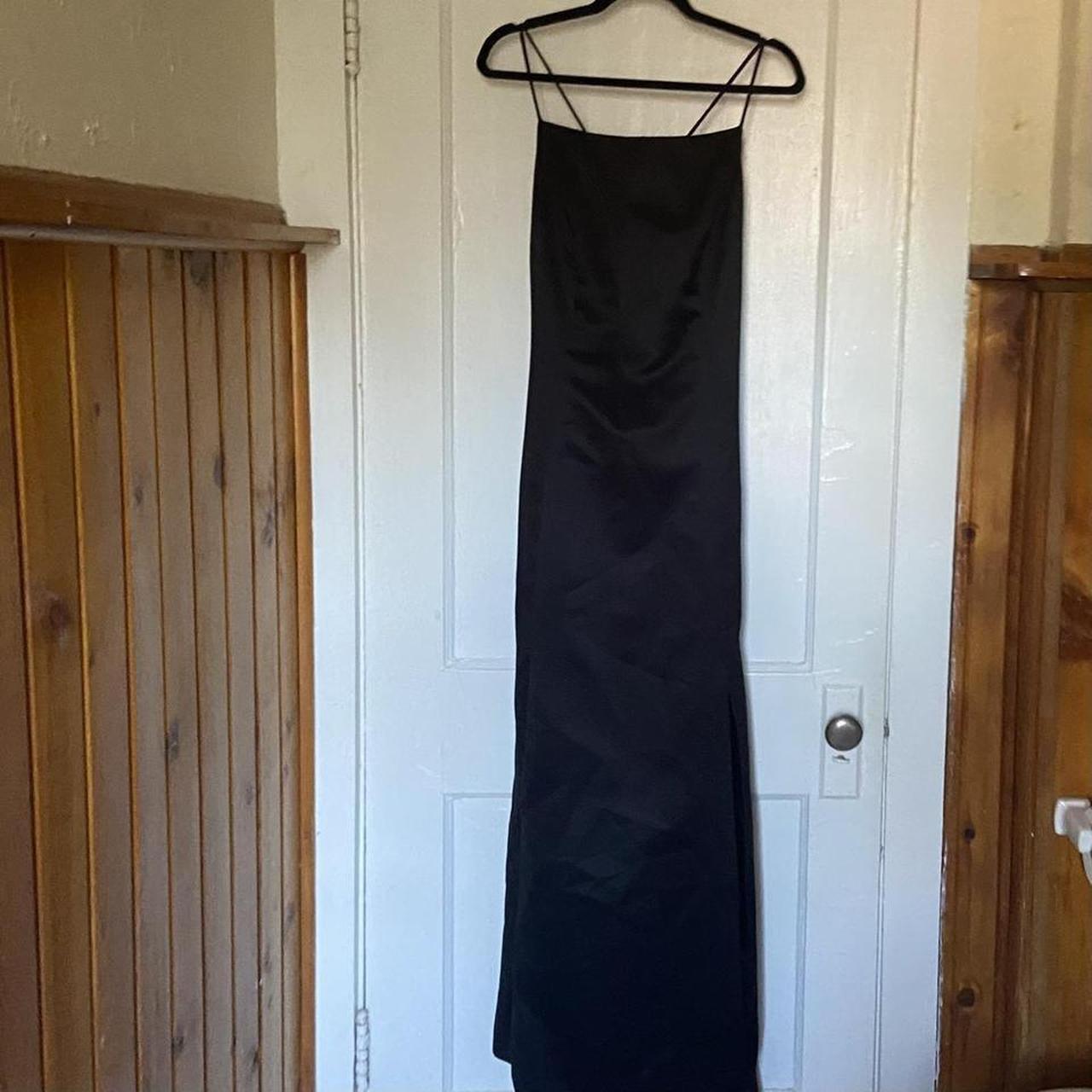The image features a black, slim-fitting, spaghetti strap dress with a silky, slinky texture, likely used as a slip. It hangs from a black hanger on the top of a slightly ajar white door, which has a round metallic knob and a keyhole beneath it. The door, featuring two rectangular panes, stands out against off-white walls with wooden vertical paneling along the bottom. To the right side of the image, a mysterious white object protrudes from the wall below the doorknob level, possibly a misplaced doorstop as the door opens inward. The scene suggests an entrance to a room, likely in a house built between the 1970s and 1990s, with color tones of brown, white, and black throughout.